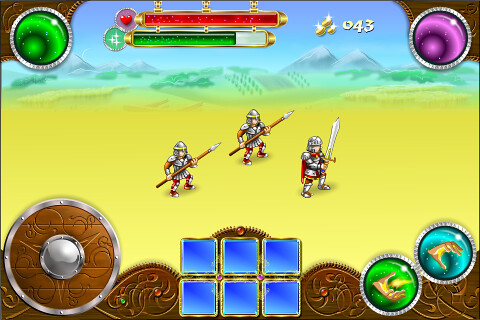In the dynamic scene of a recent mobile game, the user interface is prominently featured. At the top of the screen, two horizontal bars display essential player stats: a red heart icon represents the health bar, while a green bar with sparkling effects signifies mana or magic. The player's current gold count, tallying at 43 pieces, is also visible. Adjacent to this, a green globe and a purple globe anchor the corners of the top UI, adding to the game's thematic elements.

The in-game environment is set in a desert, where three knights clad in armor are positioned—two brandishing spears and one wielding a sword. At the bottom, additional UI elements include a shield icon, six blue boxes centrally aligned, and two circles on the lower right. These circles feature hands making different gestures, presumably for interacting with or commanding the knights. The combination of these elements suggests a rich, interactive gameplay experience characteristic of a modern, microtransaction-based mobile game.